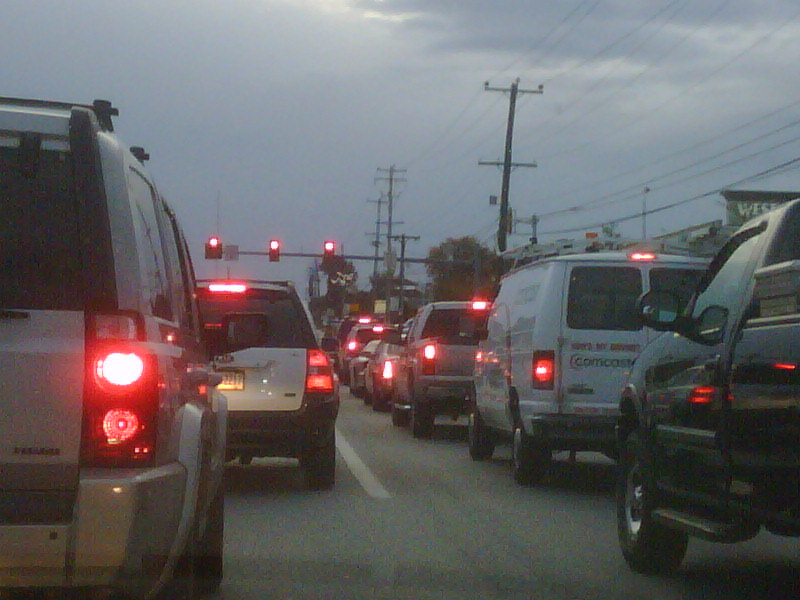This color photograph, taken from the perspective of a person inside a vehicle, shows a scene of bumper-to-bumper traffic extending into the distance. The viewpoint suggests the photographer is in the left lane, possibly leaning out from the passenger side. To the right, a line of cars stretches out, their red brake lights illuminated, indicating they are stopped at a red traffic light.

The sky, a dark blue with patches of grayish-blue clouds, suggests the time is around dusk. Above the road in the distance, three horizontally aligned traffic lights are visible, each with its red circular LED light illuminated, explaining the halt in traffic. The lanes are divided by intermittent solid white lines, separating the car rows on both sides.

On the right-hand side, power poles with thin black wires, likely for telephone and electrical lines, line the road, giving the scene a sense of urban infrastructure. Additionally, the edge of a gray building, part of a shopping area or a hotel with a partial sign reading "West," can be seen. The variety of vehicles visible includes silver, white, black, and dark blue cars, all contributing to the congested traffic scene.